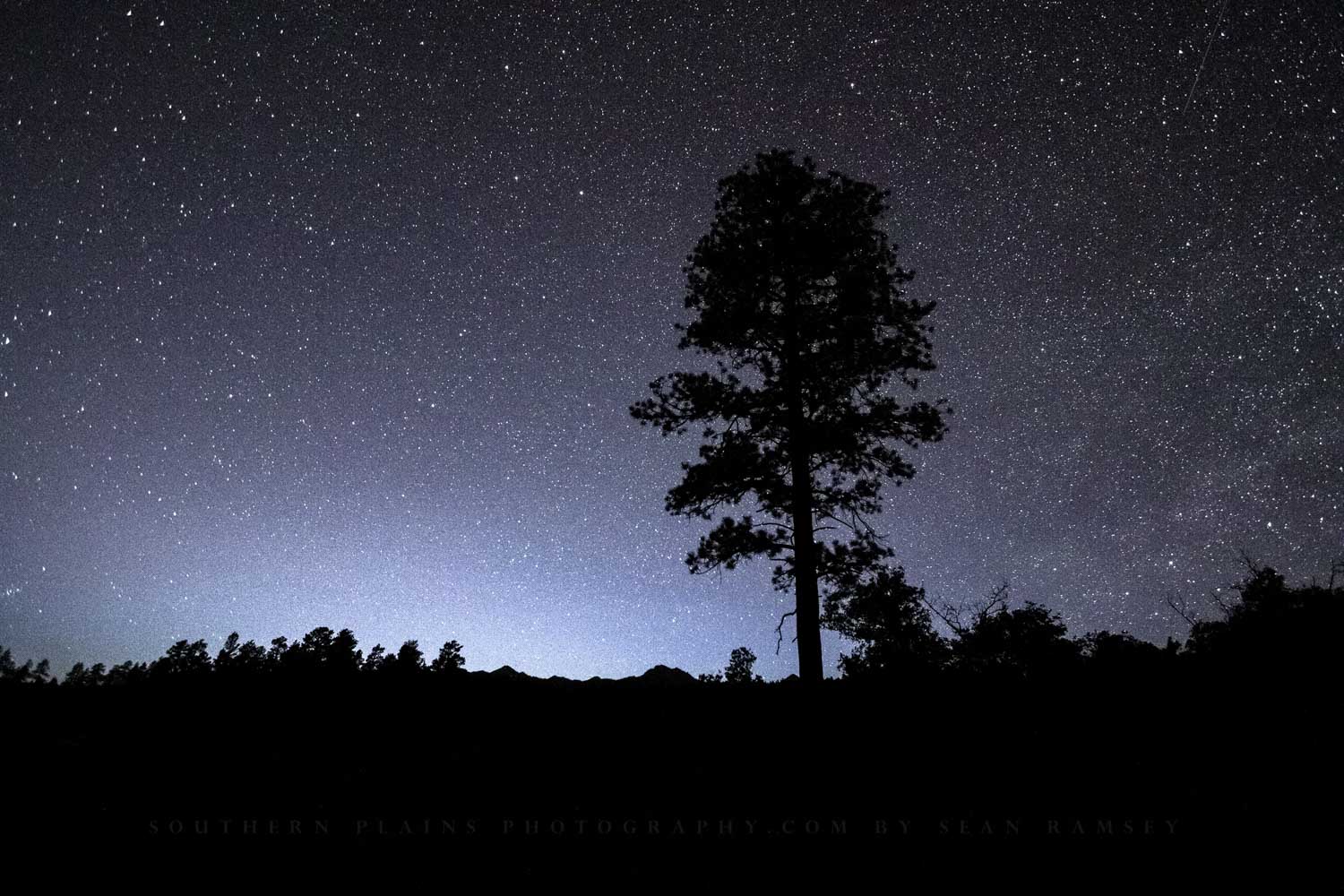In this striking nighttime photograph, a tall, thin silhouette of a large tree stands prominently against a deep midnight blue sky. The upper two-thirds of the image are peppered with countless tiny white stars, creating a sense of vastness and the appearance of the Milky Way. The horizon at the bottom glows with a light bluish hue, transitioning into darker shades of purple and black as it ascends. Small bushes and hillside vegetation can be faintly seen below the tree, although they are nearly indistinguishable in the night. This ethereal scene is illuminated by a mysterious glory light emerging from the ground, possibly from the moon, distant sunlight, or even a vehicle, enhancing the serene yet awe-inspiring beauty of the landscape. The contrast of the completely black tree silhouette with the star-studded sky captures the mystique and tranquility of the natural night.